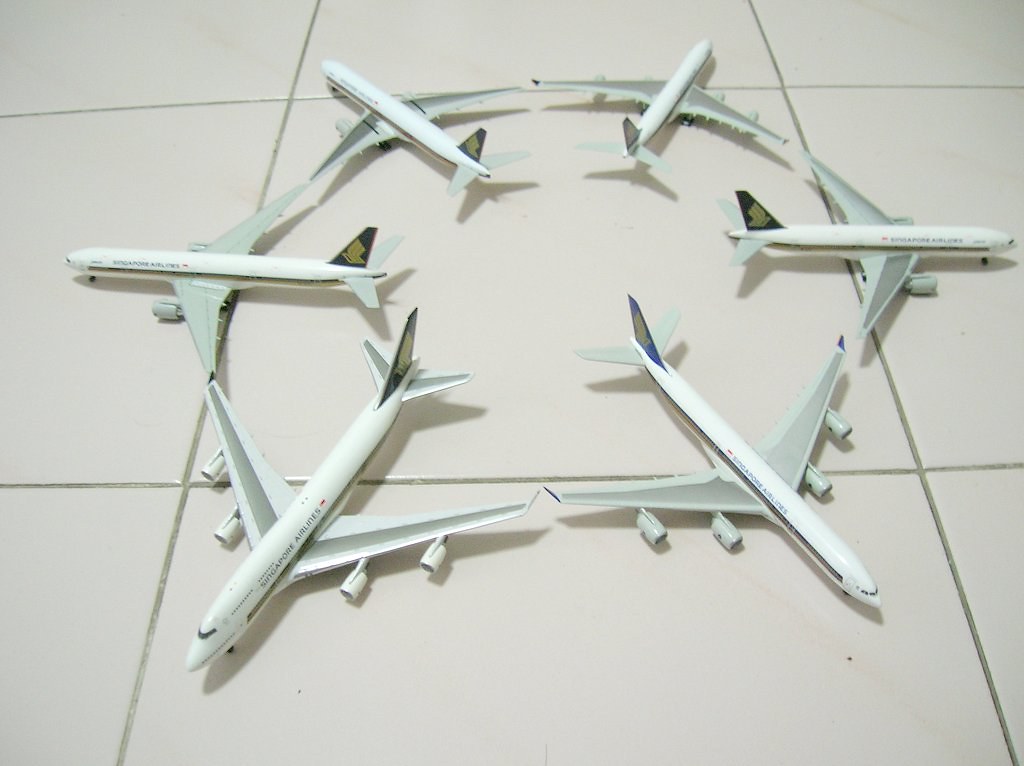In the center of the image, six model airplanes are meticulously arranged in a circular or hexagonal formation on a large, white tiled floor with dark grout, suggesting prolonged use. The tiles exhibit a faint hint of pink or other subtle colors. Each model airplane, uniform in design, represents a Singapore Airlines passenger jet, characterized by its white main body, gray wings, and blue tail fins adorned with a yellow, stylized logo. The airline's name, "Singapore Airlines," is prominently displayed in blue writing along the side of each plane, with a Singaporean flag near the tail. The airplanes' wingtips touch, forming a seamless geometric shape, with their tails all converging towards the center. Notably, while most airplanes have two engines, a few possess four engines, adding a slight variation to the otherwise identical fleet.